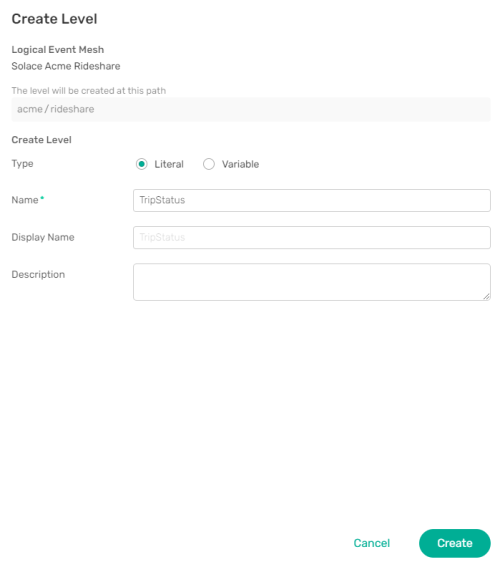This screenshot captures an interface from unidentified software, prominently featuring a page titled "Create Level." Directly below the primary heading, a subheader reads "Logical Event Mesh Solace Acme Rideshare," though the meaning of these terms is unclear.

Further down, the text "The level will be created at this path: Acme/Rideshare" is displayed in lighter font, suggesting it is a descriptive note. Another section titled "Create Level" follows, featuring the label "Type" with two options: "Literal" and "Variable." The "Literal" option is currently selected, indicated by a filled green dot in the corresponding radio button.

In the "Name" field, marked as required by a green star, the text "trip status" is entered. Subsequently, fields for "Display Name" and "Description" are present, although their contents are not specified in the screenshot. This detailed capture provides insight into the structure and options available within this software's "Create Level" function.